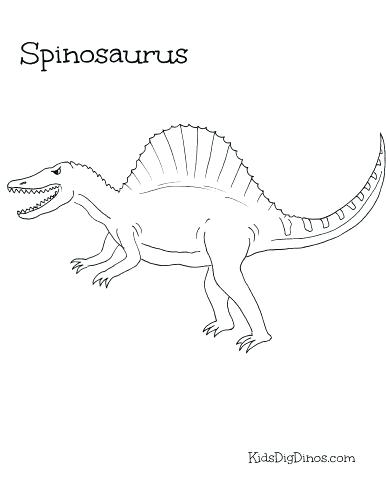This black-and-white image, designed in the style of a children's coloring book, features a Spinosaurus prominently centered on a completely white background. The name "Spinosaurus" is written in playful, kid-friendly black thin text at the top. In the bottom right corner, in smaller black writing, is the website name "kidsdigdinos.com." The dinosaur is standing on its hind legs facing left, with its mouth wide open, revealing many sharp teeth. It has angry-looking eyes and short, muscular arms with three clawed toes. The Spinosaurus has large, muscular back legs and a thin, striped tail extending to the right. Its back is adorned with a tall, jagged fin running from its neck to its tail, reminiscent of its spinous process. While the image is not overly detailed, it effectively captures the creature’s fierce and imposing appearance, making it suitable for educational or children's activity books.